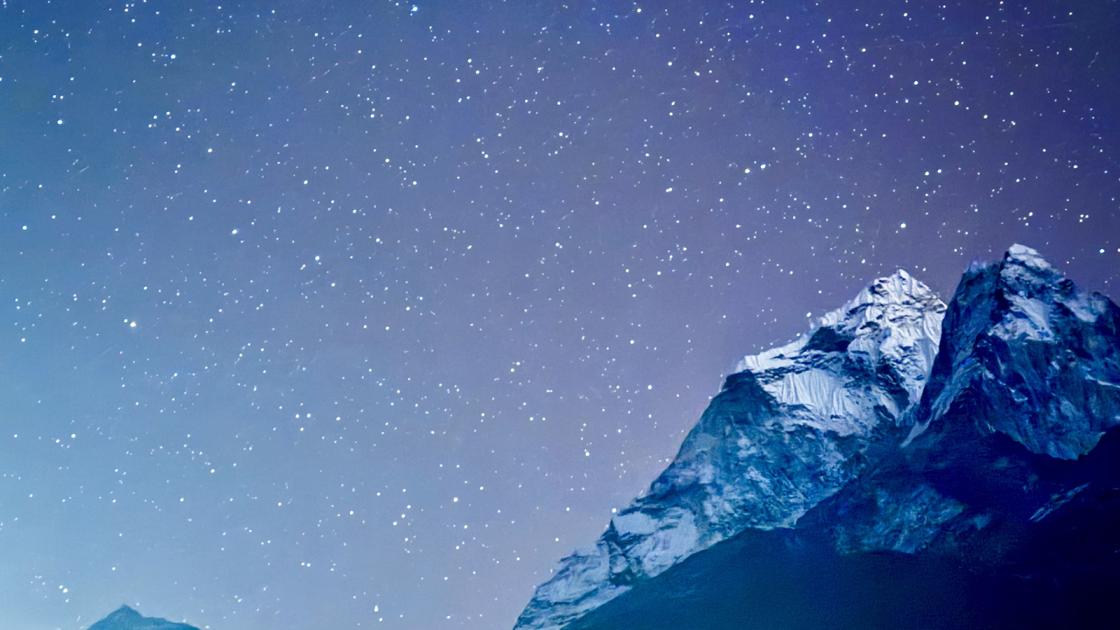The photograph captures a breathtaking, professional shot of a craggy, mountainous landscape under a captivating night sky. On the right side of the frame, sharp, rugged mountain peaks, possibly composed of stone or granite, are bathed in shades of cold blue and silvery light, creating a stark contrast against the deep, dark shadows. The mountainous terrain extends to the lower left corner of the image, revealing just a small peak. The expansive sky, which dominates the majority of the frame, is filled with a myriad of white stars set against gradients of deep blue, whitish gray, and a purplish hue to the right. The entire scene is illuminated by what appears to be moonlight, lending a brighter, almost ethereal quality to the central portion of the sky, reminiscent of the Milky Way's glow. The detailed, icy-looking textures of the mountains evoke a sense of freezing cold, adding to the photo's Northern or Arctic ambiance, despite the absence of any snow or ice.